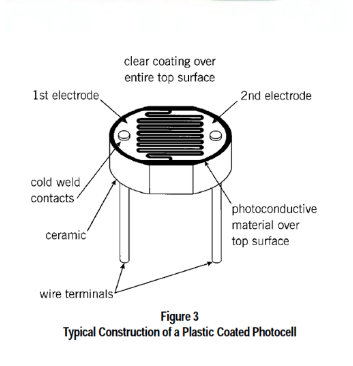This black and white illustration, likely from an instructional or educational source, is titled "Figure 3: Typical Construction of a Plastic-Coated Photocell." The central image depicts an elongated, can-shaped photocell with two wire terminals protruding from the bottom. Various components are labeled with black text and arrows pointing to specific parts of the device. The top of the photocell features a grill-type element with two screws, marked as "cold-weld contacts." Surrounding the flat top surface are labels like "clear coating over entire top surface," "first electrode," and "second electrode," with some directed at the flat part itself. The outer casing is identified as ceramic, while the "photoconductive material over top surface" is also indicated on the flat area. Wire terminals are highlighted at the bottom by two arrows. This detailed diagram is a quintessential example of what one might encounter in a product manual or textbook, elucidating the construction of a plastic-coated photocell.